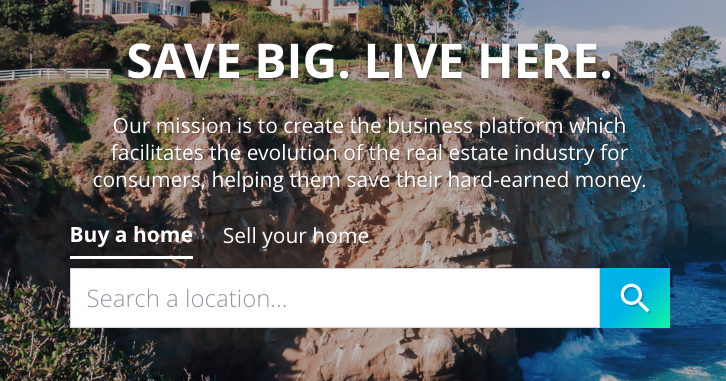This digital graphic for a real estate platform prominently features the slogan "Save Big, Live Here" in bold lettering. The background image showcases a serene cliffside landscape with rocky formations, blue waters, and lush greenery, including grass and shrubs. In the distance, a collection of houses, predominantly red brick with one featuring white siding, are nestled amidst trees and shrubs under a blue sky dotted with clouds. A white wooden fence can be seen on the far left, while a paved walkway appears on the far right. The platform's mission statement, "Our mission is to create the business platform which facilitates the evolution of the real estate industry for consumers, helping them save their hard-earned money," is clearly displayed. The interface includes a search bar labeled "Search Location" on a white background with grey lettering, accompanied by a blue magnifying glass icon in the right corner for easy navigation.